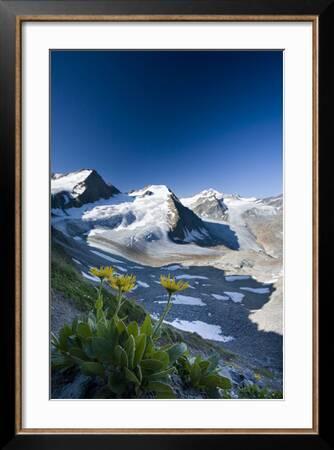The framed picture displays a serene high-altitude landscape. Encased in a stylish black frame with a gold inner lining and a thick white mat, the artwork showcases a predominantly blue pitcher capturing the tranquil scene of snow-covered mountains. In the foreground, three vibrant yellow dandelions with lush green leaves thrive despite the wintery surroundings, signifying resilience against the cold at such elevations, likely between 8,000 and 10,000 feet. Mid-image, a rocky field interspersed with patches of snow and pools of water stretches out, adding a contrasting texture to the scene. Above, the sky transitions from a deep navy at the top to a lighter shade of blue towards the bottom, enhancing the peaceful ambiance of the natural setting.